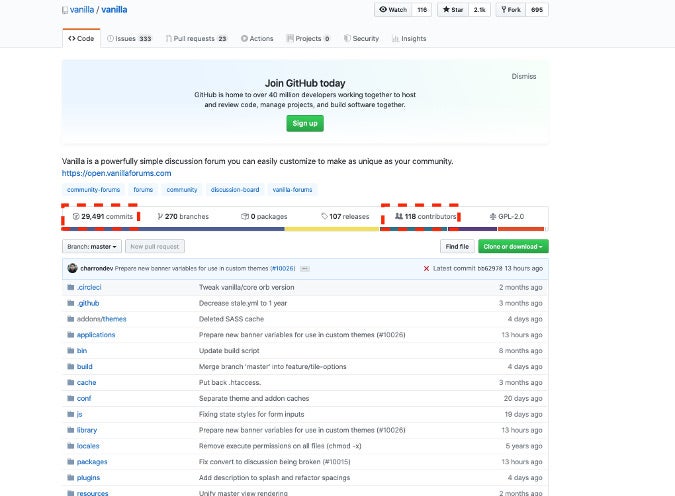The image depicts a screenshot from a website, centered around the branding for "Vanilla." The website’s logo appears at the upper left-hand side, displaying the name "Vanilla" two times, one written in lighter blue beside a small cell phone icon, followed by a slightly darker blue "Vanilla." On the top right-hand corner of the screen, a navigation menu is visible.

Below the logo and navigation menu, several tabs are aligned horizontally. These inclusively list:
- Code
- Issues
- Requests
- Actions
- Projects
- Security
- Insights

Following these tabs, there is a prominent banner urging visitors to "Join GitHub Today." This banner features two actionable elements: a "Dismiss" button located in the upper right corner and a "Sign Up" button situated at the bottom center of the banner.

Under the banner, a descriptive text highlights the platform's value proposition: "Vanilla is a powerful, simple discussion forum you can easily customize to make as unique as your community." Beneath this, there is a URL directing to a Vanilla forum web address, and below that, a list of items is presented, though the specific content of this list is not detailed in the description.